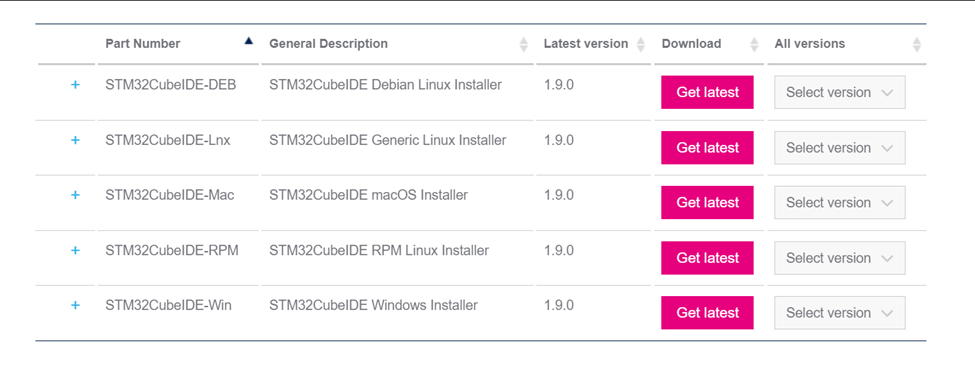This image is a screenshot depicting a detailed table of parts. The table is structured into five columns: "Part Number," "General Description," "Latest Version," "Download," and "All Versions." Each row is dedicated to a different part or item, detailed under these categories.

- **Part Number**: Each part's identifier. To the left of each part number, there is a blue plus sign.
- **General Description**: Provides a more in-depth description, including the part number.
- **Latest Version**: Indicates the most recent version available for each part, which is consistently version 1.9.0 across all parts.
- **Download**: Contains a red button with white text for downloading the parts.
- **All Versions**: Features grayish-white dropdown boxes with a small arrow for selecting different versions.

The table and its contents are set against a completely white background. Organizing its layout, there are two horizontal gray lines—one positioned above and the other below the table. The origin of this table, whether from a particular website or software, is indeterminate based on the screenshot alone.